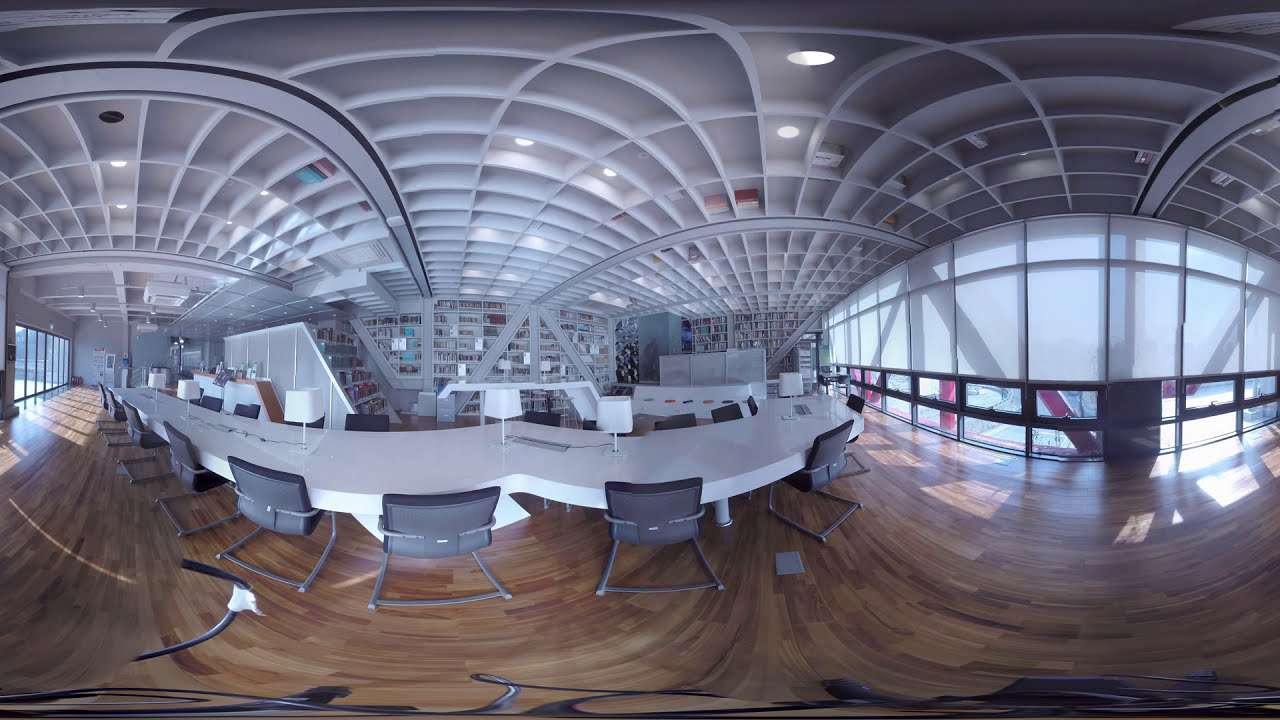This panoramic image captures the interior of a spacious, modern room, with notable lens distortions that create an intriguing perspective. At the heart of the image is a lengthy, white rectangular table, accompanied by a combination of standard black chairs. The table features an unusual curved extension, giving it a unique U-shape at one end. Scattered along the table are white table lamps, enhancing the modern aesthetic.

The room's floor is a patchwork of different shades of wooden planks, adding warmth and texture to the space. The ceiling, though distorted to seem arched due to the fisheye lens, is actually flat and white, embedded with lights that blend seamlessly into the design.

Dominating the background are extensive white bookshelves, partially filled with various books and other items, creating a library-like atmosphere. Situated between these shelves and the long table is an additional set of stair-like shelves, adding depth and visual interest.

Natural light floods the room from rows of vertical windows on both the left and right sides. The windows are partially covered with slightly translucent curtains, allowing soft light to highlight the floor while revealing the shadows of structural elements outside. On the right, more visibility is granted through the lower windows, revealing red structural columns outside. This intricate balance of artificial and natural lighting creates a bright, inviting environment.